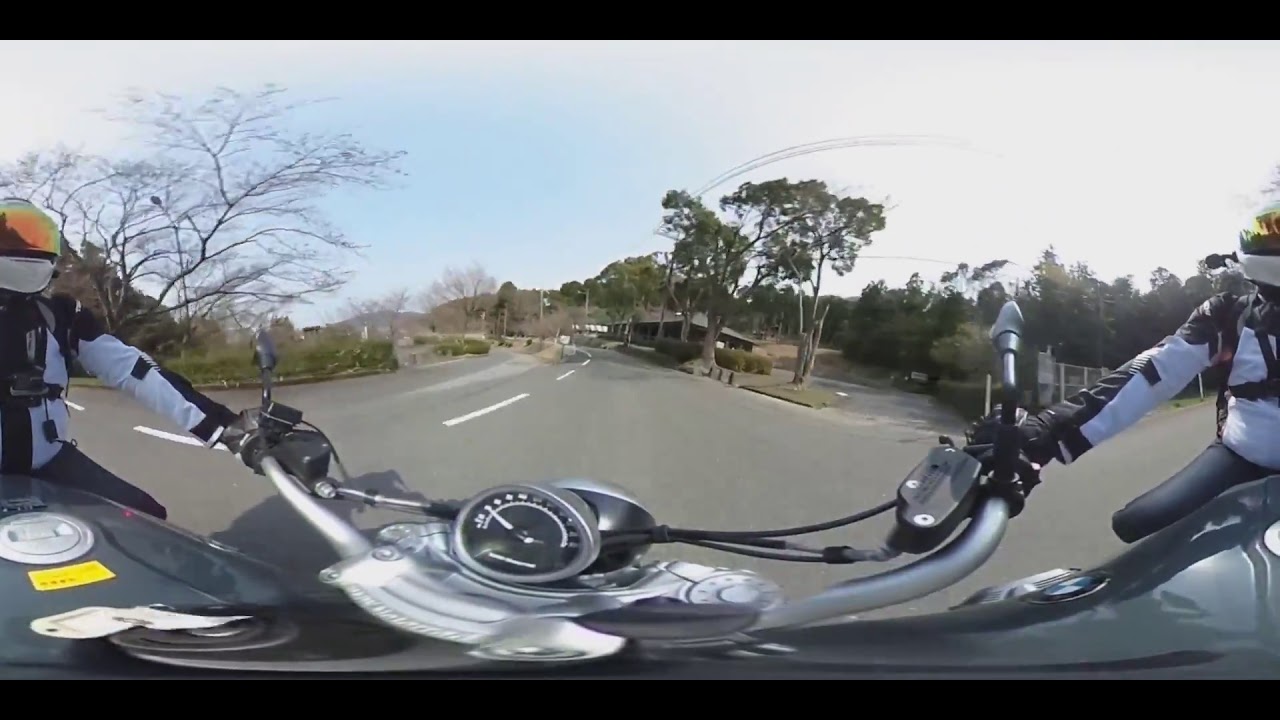The photograph, likely taken with a wide-angle or panoramic lens, offers a dynamic view from the perspective of a motorcyclist. The distortion effect curves the scene, making the image both captivating and immersive. In the foreground, the motorcycle's handlebars and an instrument panel, featuring a white-dial speedometer on a black background with unreadable numbers, dominate the view. A small BMW emblem is visible on the handlebar. The rider, clad in a black and white jacket and black pants, grips the handlebars. They also wear a helmet with a yellow visor. The motorcycle appears black in color.

They are traveling down a two-way road marked with a broken white dividing line. To the right, lush trees full of leaves border the road, along with a fence and a structure that may be a building or rest stop. On the left, a solitary tree stands leafless, suggesting a season like fall or winter. There is also a yellow sign visible to the left of the handlebar, though its text is unreadable. The sky is both sunny and bright, with a mix of overcast high clouds and patches of blue. Overall, the photograph captures a moment of motion and adventure on a scenic route.